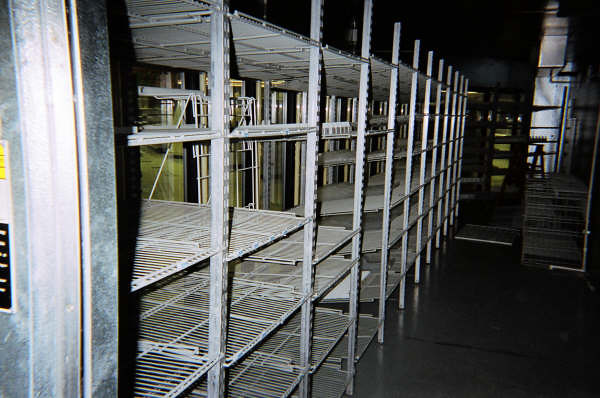This image depicts a large stainless steel shelving unit, possibly situated in a warehouse or industrial setting. The shelving, which consists of robust metal supports and thin metal tubes forming the shelves, stretches horizontally across the left half of the image, extending into the distance. The unit appears to have four or five tiers and is approximately 20 sections deep. In the foreground, there is a prominent stainless steel pillar adorned with a sticker. The low lighting obscures the ceiling and background details, but additional stainless steel structures and shelving units are faintly visible. The floor beneath is black, and there's a hint of yellow lighting in the distance, adding a dim glow to the scene. The overall ambiance suggests an expansive storage area designed for heavy-duty use.